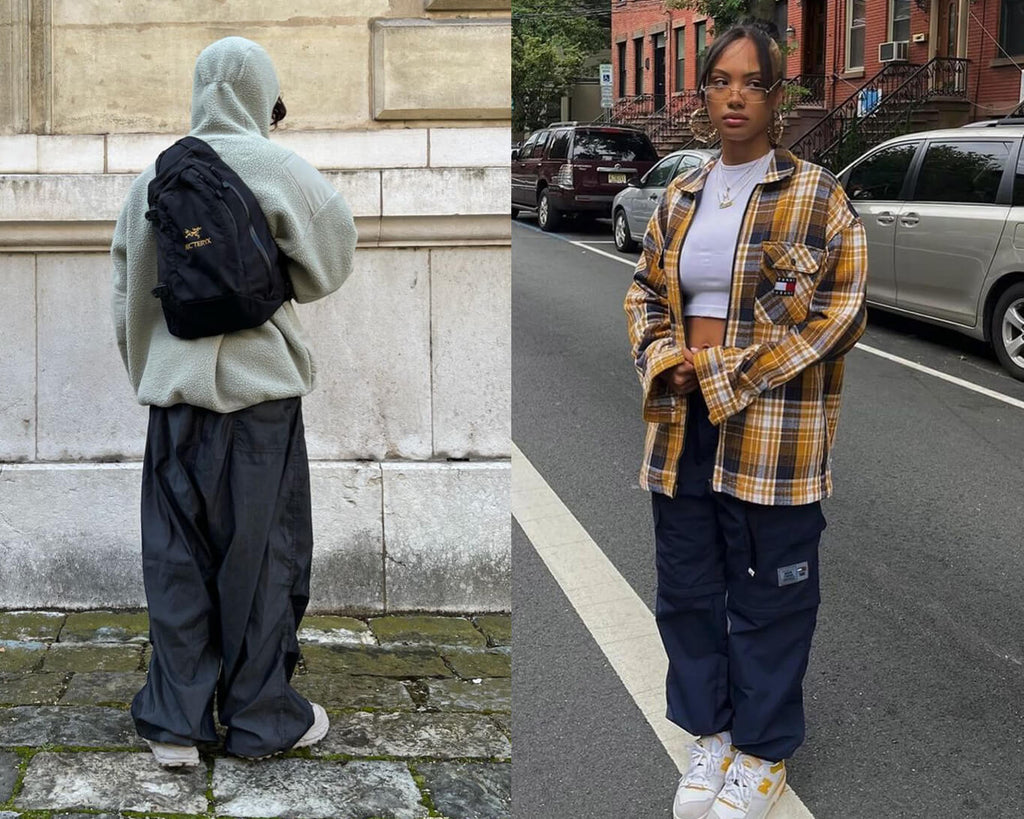The combined image is a split diptych juxtaposing two distinct scenes. 

On the left, a person stands with their back to the camera in front of an aged, grimy building. The building is composed of large white blocks at the bottom and tan blocks at the top, stained with black dirt near the edges. The ground beneath is a once-white cobblestone or brick sidewalk, now marred with green moss and black dirt. The individual wears a white hoodie with the hood up, baggy gray pants, and a black backpack.

The right side of the image features a black woman standing in the middle of a road. Behind her, a row of cars is parked in front of a brick building. She is dressed in a white crop top paired with an open plaid jacket in yellow, blue, and white, and baggy blue pants. She completes her look with thin-framed glasses and white shoes accented with orange.